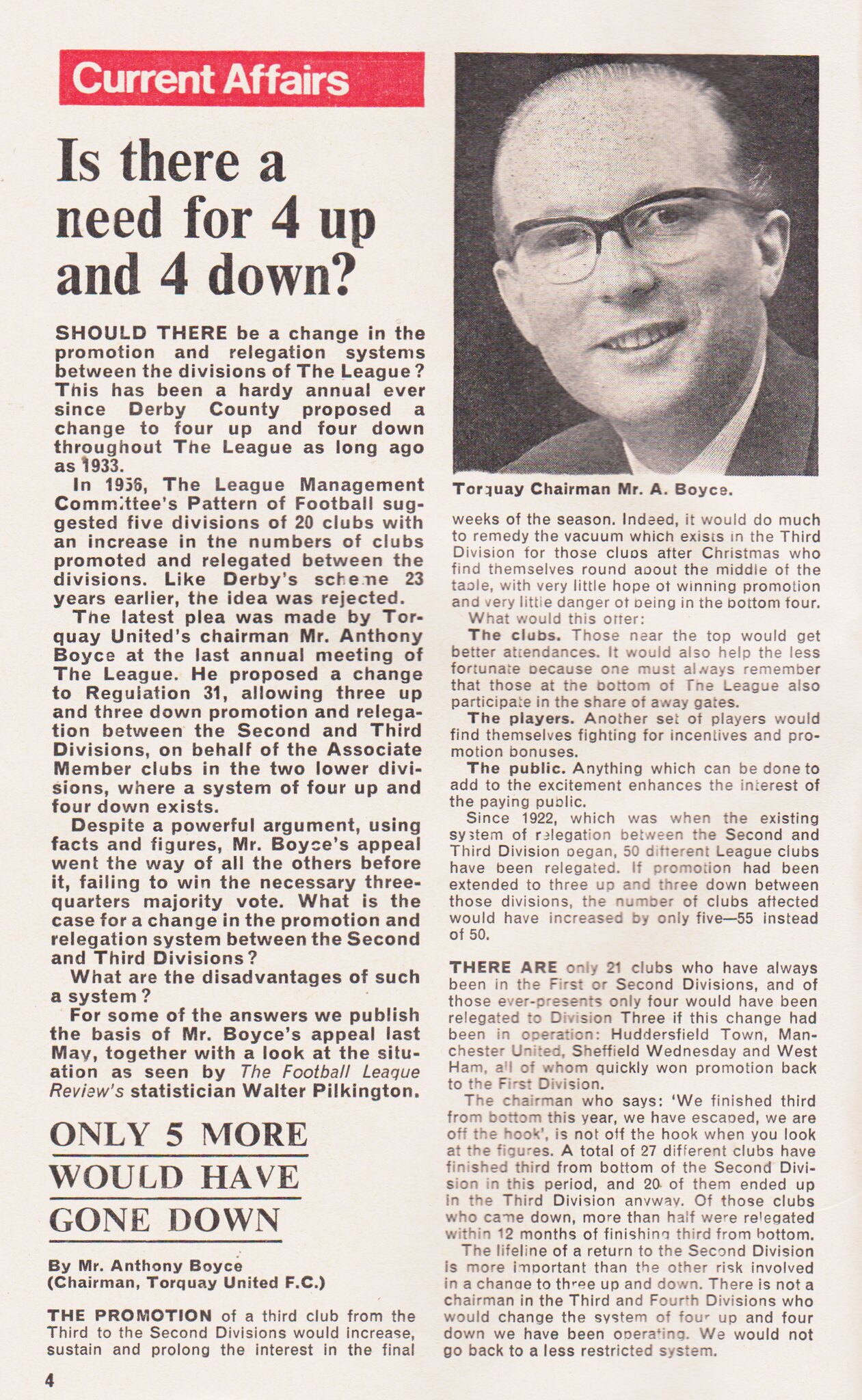The image depicts a scanned photocopy of a newspaper article titled "Current Affairs" in red text, the only color amidst a black-and-white layout. To the right of the title is a photograph of a man wearing a suit and glasses, with the caption beneath it identifying him as Torquay United's Chairman Mr. Anthony Boyce. The headline underneath the "Current Affairs" title reads, "Is there a need for four up and four down?" The article debates proposed changes to the British football league's promotion and relegation system, citing historical proposals and arguments, including Mr. Boyce's recent proposal at the league's annual meeting. Despite his compelling case for transitioning to a three up, three down system between the second and third divisions, similar past attempts have been unsuccessful. The article includes detailed statistics and arguments highlighting the potential benefits of such changes to both clubs and public interest, while also noting the challenges in achieving the necessary majority vote for these changes. At the bottom of the page, in all caps and underlined, the text reads, "Only five more would have gone down."